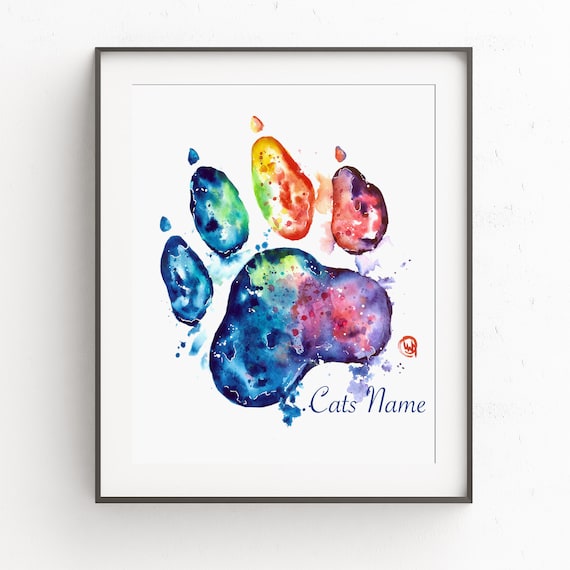The product image features a framed watercolor print of a cat's paw, meticulously detailed and artistically vibrant. The frame is thin and comes in a silver or dark grey finish, adding a sleek touch to the overall aesthetic. The painting is set against a thick white matte, enhancing its prominence. The cat's paw, tilted slightly to the left, showcases an array of colors including blue, purple, green, red, and orange, with each toe bean and fingernail uniquely tinted. Above the paw, the toenails have distinct nail prints visible. Beneath the paw, there is customizable cursive text reading "cat's name," indicating a placeholder for personalization. Additionally, a small red circle with the artist's initial is positioned to the right. The artwork includes a thin white border inside the frame, providing a clean and elegant presentation. This detailed and vibrant print is perfect for proud cat owners looking to add a personalized touch to their decor.